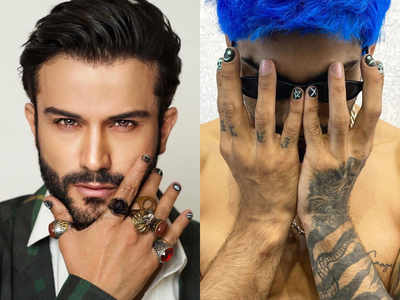The image features a split-screen composition of two headshot-style portraits, each showcasing a different man who might possibly be the same individual due to distinct similarities. On the left, the man has dark brown or black hair that is meticulously styled, swooped back, and combed over, drawing attention to his striking features, including a well-defined jawline and neatly trimmed beard. He holds his hand up to his face, prominently displaying several gemstone signet rings on his fingers. His nails are painted black with an iridescent accent, adding to his well-groomed appearance. He is dressed in a green suit with a white dress shirt, though the lower parts of the outfit are out of frame.

On the right, the second image depicts a man with vibrant blue hair, reminiscent of Milhouse from The Simpsons. He is holding his face with both hands, obscuring much of his facial features but revealing slim sunglasses and several tattoos on his fingers and forearms. His nails feature a similar design to the first man’s, further suggesting they might be the same person. He appears to be shirtless, but his hands strategically cover his chest, ensuring modesty. This portrait contrasts with the first, with a more candid and casual quality compared to the well-composed look on the left.